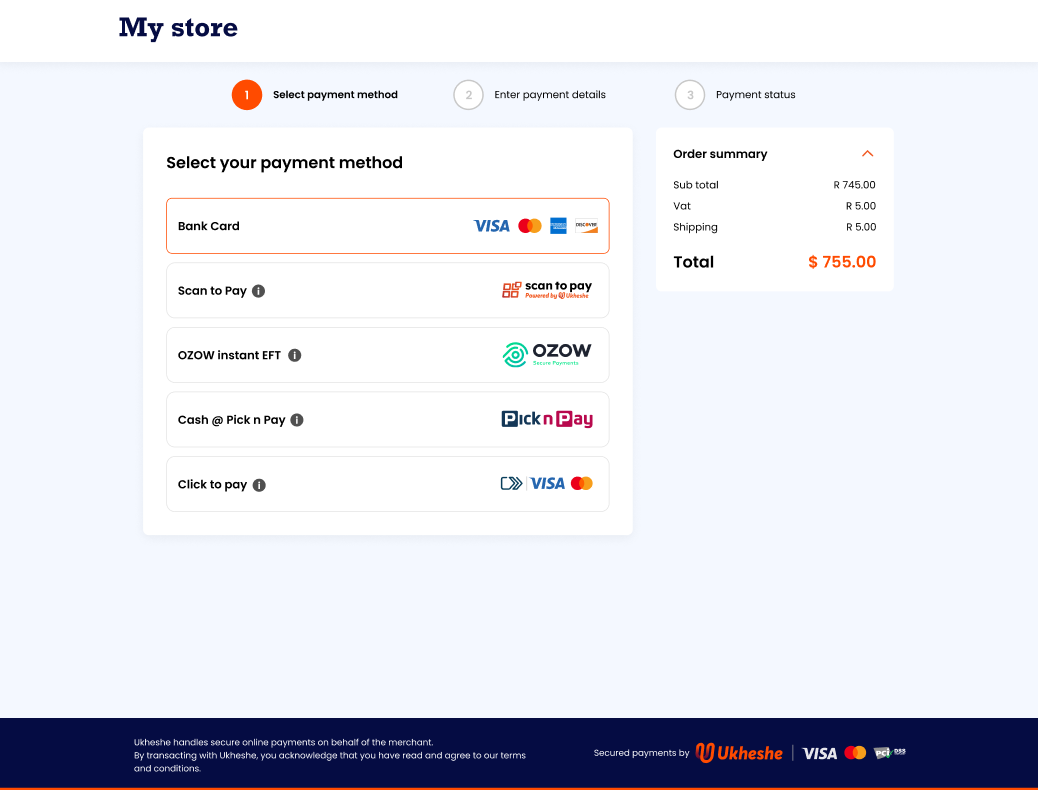The image features a clean, light blue background with various elements designed for an online payment interface. At the top, a white box displays "My Store" in blue text. Below this, a prominent red circle with the number "1" indicates the step "Select Payment Method." This is followed by a smaller red circle with the number "2" labeled "Enter Payment Details," and another with the number "3" marked "Payment Status."

Further down, a white box reads "Select Your Payment Method" and lists options like Bank Card, Visa, MasterCard, American Express, and Discover, with a slightly outlined red box highlighting the selection. Just below, there's a section labeled "Scan to Pay" accompanied by a gray circle with an information icon.

The image also includes other payment options such as OZAL Instant EFT with a gray exclamation point, and "Cash at Pick and Pay" highlighted with a gray information icon. The right side features the Pick and Pay logo in blue and pink, along with Click to Pay instructions and a blue arrow pointing right, followed by Visa and MasterCard icons.

On the far right, a white box labeled "Order Summary" provides a breakdown of costs, with a red arrow pointing upwards showing the Subtotal at $745, VAT at $5, Shipping at $5, and a Total of $755 in red.

At the bottom, a large dark blue box outlined in red contains some text, with "U" and "UCashE" in red, and a smaller white box displaying Visa and MasterCard logos.